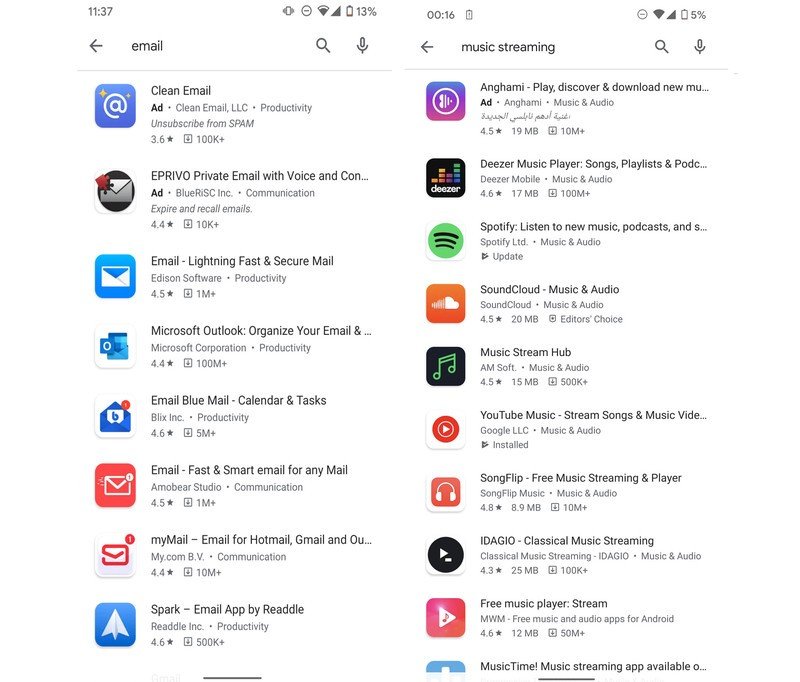The image captures a side-by-side comparison of two screenshots on a mobile phone, meticulously aligned to create the illusion of a twin picture. The left screen displays a selection of email applications listed vertically, starting from "Clean Email" at the top, followed by "ePrivo Private Email with Voice & Contact," "Email - Lightning Fast and Secure Mail," "Microsoft Outlook - Organize Your Email," "Blue Mail - Email, Calendar & Tasks," "Email - Fast & Smart Email for Any Mail," "myMail - Email for Hotmail, Gmail, and Outlook," and ending with "Spark Email App by Readdle."

On the right screen, a variety of music streaming apps are showcased, including "Anghami," "Deezer Music Player," "Spotify," "SoundCloud Music & Audio," "Music Stream Hub," "YouTube Music," "Songflip," and "Audiomack Free Music Player." The bottom of the screen cuts off, suggesting there are additional apps not fully visible in the image.